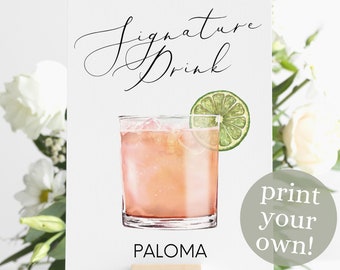The image features an aesthetically arranged advertisement for custom printing. Central to the composition is a white card displaying a cocktail illustration. The drink appears in a rocks glass, filled with a pink, peach-colored liquid, and garnished with a slice of lime on the rim. Above the glass, in black cursive script, are the words "Signature Drink," and below, in bold black capital letters, it reads "PALOMA." Adjacent to this illustration is a gray circle adorned with the text "PRINT YOUR OWN!" in white print. The background adds to the visual appeal with a serene arrangement of white roses, white daisies, green baby's breath, and other greenery set against a white wall, enhancing the artistic and inviting nature of the advertisement. This elegant setup suggests a promotional concept for creating personalized drink labels.